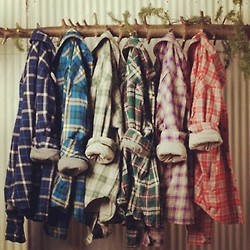The image depicts a textured white wall adorned with a tangible striped pattern. Mounted horizontally across the wall is a rustic, wooden tree branch serving as a coat rack. Green leaves sporadically sprout from the branch, indicating its natural origin. Seven flannel shirts in various plaid patterns are neatly hung from hooks along the branch. Each shirt's left sleeve is rolled up. The shirts, from left to right, are: dark blue and white plaid, lighter blue with red plaid, white and light green plaid, a Christmas-themed green, red, and white plaid, pink, purple, and white plaid, and finally, a red and beige plaid. The scene resembles a curated display, likely in a retail store.